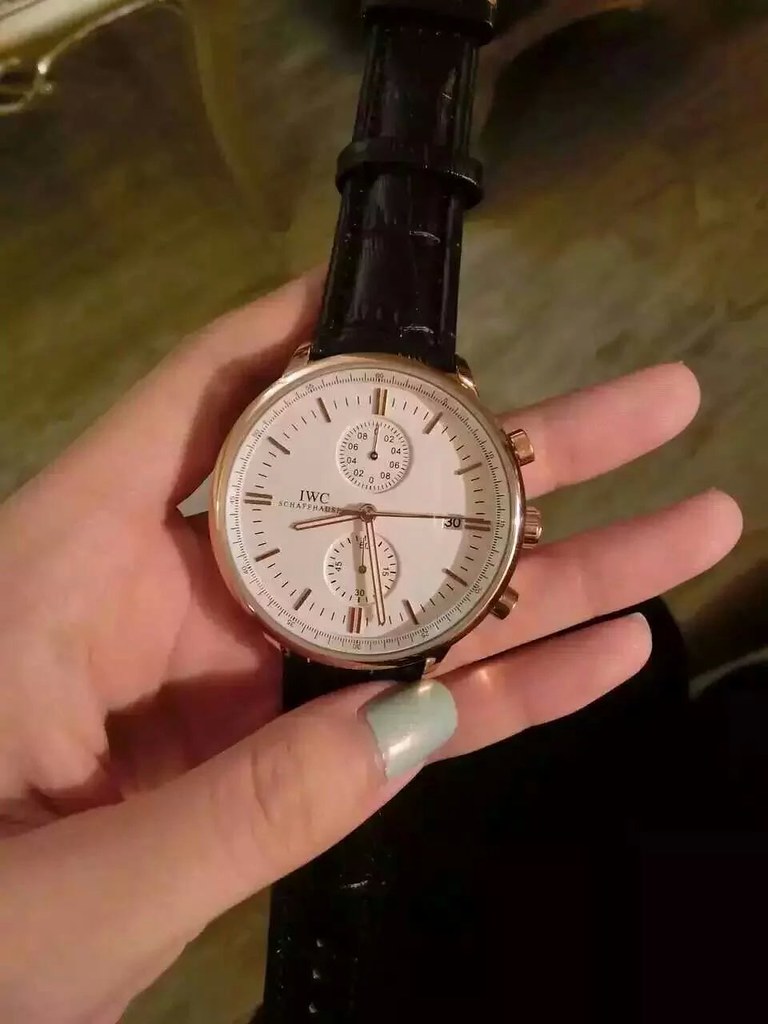The image showcases a close-up of a wristwatch being held in the open palm of a Caucasian woman's hand, characterized by long, slender fingers and nails painted in a light jade green. The watch features a round face with a gold bezel and a white dial interior. It lacks traditional numerical hour markers, instead displaying double hashes for the main hour positions (12, 3, 6, and 9) and single hashes for the remaining hours, along with minute markers in-between. The watch hands, which are copper-toned, indicate a time of approximately 8:28. The face of the watch also includes two smaller sub-dials, one located just below the 12 o'clock position and another above the 6 o'clock position, though their exact functions remain unspecified. The wristwatch is secured with a black leather band, which has a textured finish resembling snakeskin or eelskin. The background of the image reveals a brown floor and a dark, indistinct object that appears to be a table on the right-hand side.